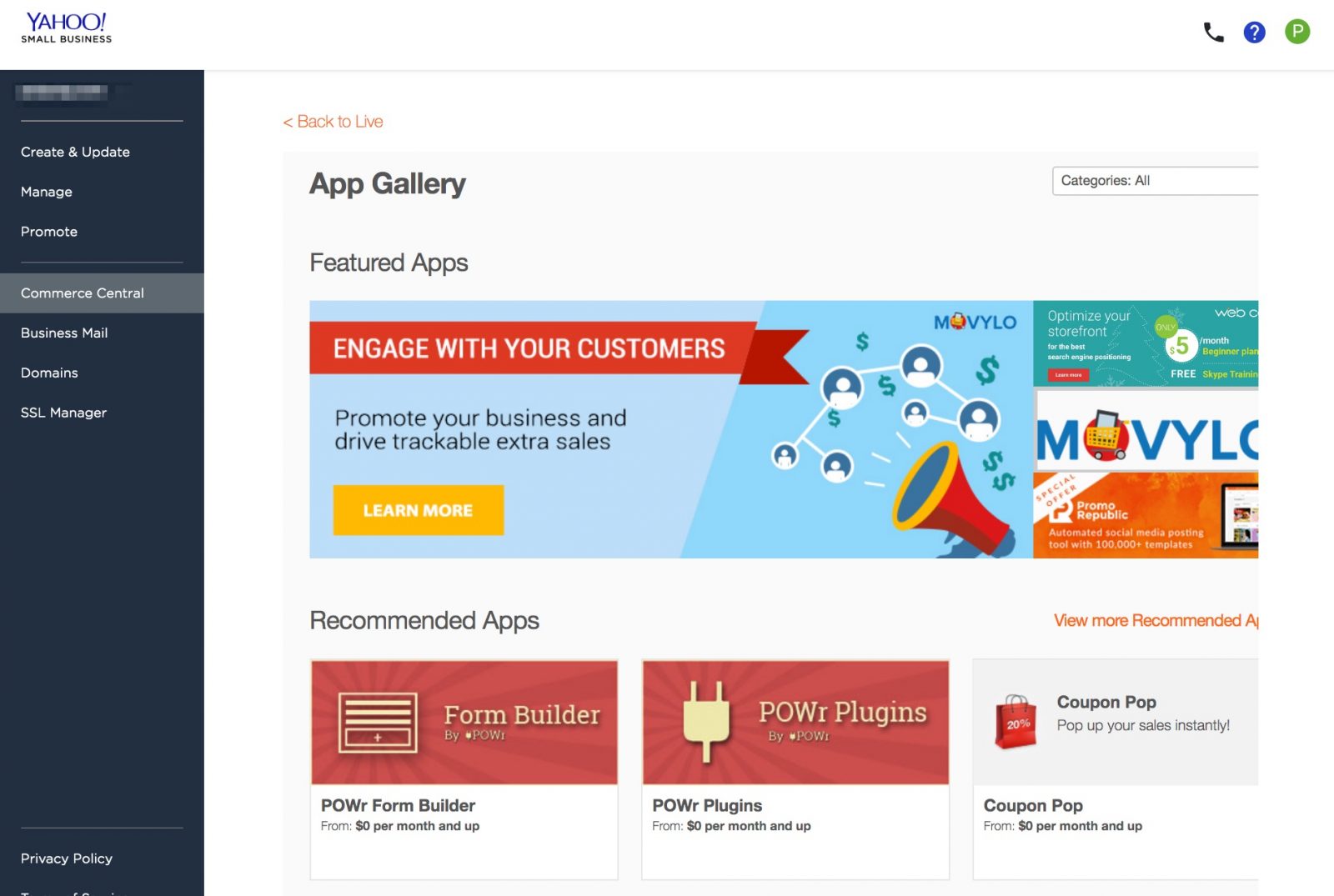This image displays a webpage interface for Yahoo Small Business. On the left, there is a navigation bar featuring various links such as "Create and Update," "Manage," "Promote," "Commerce Central," "Business Mail," "Domains," and "SSL Manager." Additional links include "Back to Life," "App Gallery," "Featured Apps," "Engage with Your Customers," and "Promote Your Business and Drive Trackable Extra Sales."

The page highlights a section encouraging users to "Learn More" about recommended applications. Prominently featured apps include "Fund Builder by POWR," starting at $0 per month, and various "POWR Plugins," which are also available from $0 per month. Another highlighted tool is "Coupon Pop," designed to "Popup Your Sales Instantly," similarly starting at $0 per month.